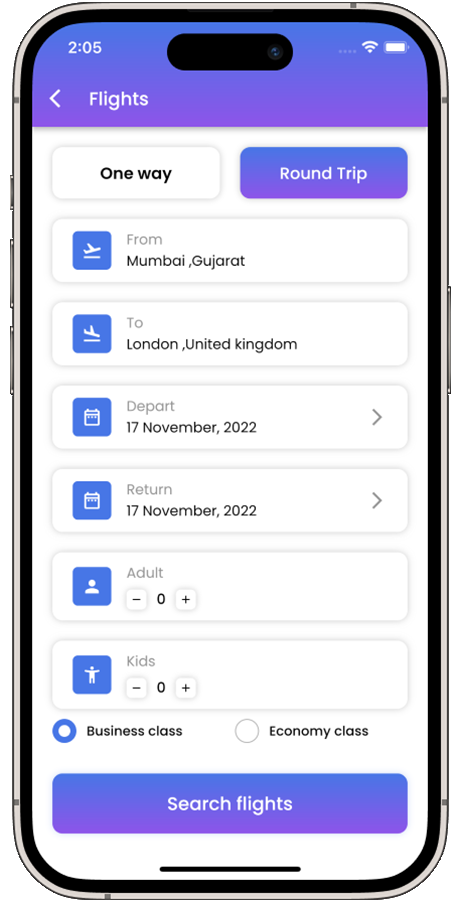The image depicts a simulated black cell phone screen. At the top, it displays the time "2:05" in white font. There is a black notch cut out for the front camera, adjacent to a white Wi-Fi icon and a white battery icon. Below this, the screen features the heading "Flights" in white text.

Two prominent boxes follow: the first is white with black text stating "One Way," while the second is purple with white text indicating "Round Trip." 

A series of white input fields fills the screen, each accompanied by various blue and white icons. The first field, labeled "From," indicates the departure location as "Mumbai, Gujarat." The second field, labeled "To," specifies the destination as "London, United Kingdom."

Next are the departure and return dates, both marked with a calendar icon. The dates listed are "17 November 2022" for both departure and return.

Another input field, blue and white, features an abstract icon of a person and states "Adults: 0, Kids: 0." Below this, two circles representing travel classes are displayed: one for "Business Class" and the other for "Economy Class." The "Business Class" circle is purple and white, indicating it is selected.

At the bottom of the screen, a conspicuous purple box with white font encourages users to "Search Flights." Beneath this button, a thin black bar is visible.